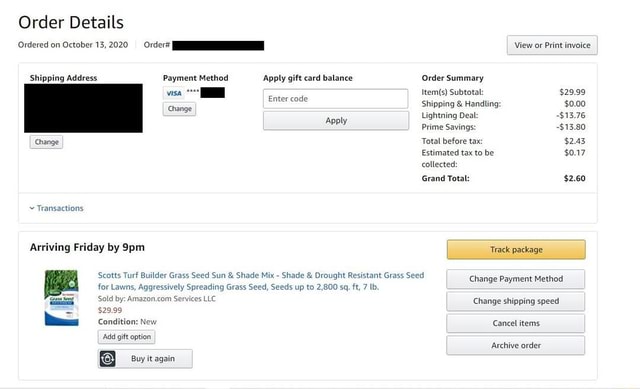The image displays an online order confirmation page, featuring various details and options:

In the top left corner, the heading "Order Details" is written in black text. Below this, the text reads "Ordered on October 13, 2020," followed by "Order Number," which is obscured by a black rectangle for privacy. On the right side of this section, there is a gray box containing the options "View" or "Print Invoice."

Continuing on the right, the "Shipping Address" section is present, but the actual address has been hidden by a large black box. Adjacent to this, the "Payment Method" section lists "Visa" followed by four tiny dots and a concealed credit card number, represented by another black rectangle.

Underneath these details is an area for applying a gift card balance, including fields labeled "Enter Code" and "Apply." 

The "Order Summary" section follows, detailing the costs: 
- Item Subtotal: $29.99
- Lightning Deal: -$13.76
- Prime Savings: -$13.80
- Grand Total: $2.60

At the bottom of the page, in a separate rectangle, it is indicated that the item is "Arriving Friday by 9 p.m." The specific product ordered is "Scott's Turf Builder Grass Seed, Sun and Shade Mix, Shade and Drought Resistant, Aggressively Spreading Grass Seed, Seeds Up to 2,800 Square Feet," listed at $29.99. To the right of this product listing, a yellow box offers the option to "Track Package."